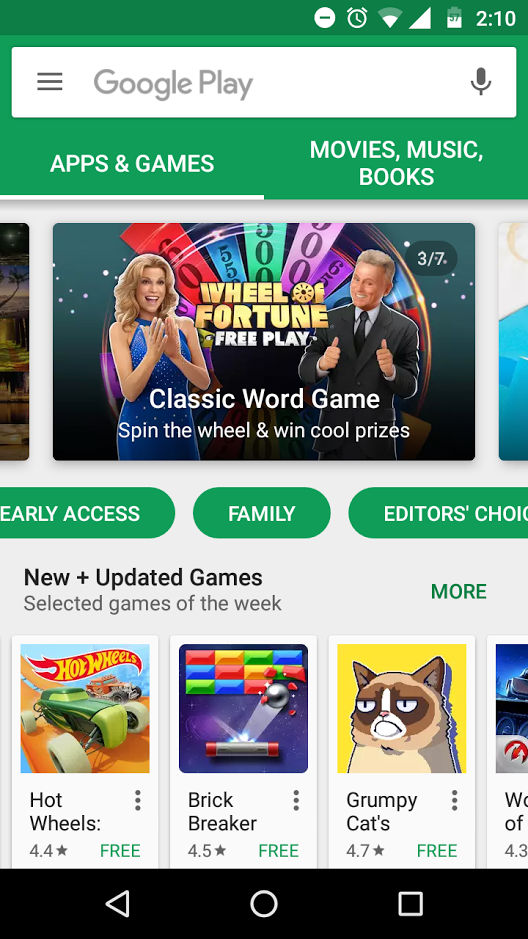This image is a screenshot of the Google Play Store for Android, captured at 2:10 PM. In the notification status bar at the top right, various icons are displayed, including the battery level at 57%, Wi-Fi signal strength, alarm clock, and the Do Not Disturb symbol.

The screenshot is focused on the "Apps & Games" category of the Play Store. Featured prominently is the game "Wheel of Fortune Free Play," a classic word game where players spin the wheel to win prizes. Below this, additional games are listed under the "New and Updated Games" section, showcasing titles like "Hot Wheels," "Brick Breaker," and "Grumpy Cats."

The Play Store interface also suggests several categories to browse through, including "Early Access," "Family," and "Editor's Choice." Furthermore, there's a mention of other media categories such as movies, music, and books. The entire interface is neatly presented in a rectangular format, typical of screenshots taken on an Android device.